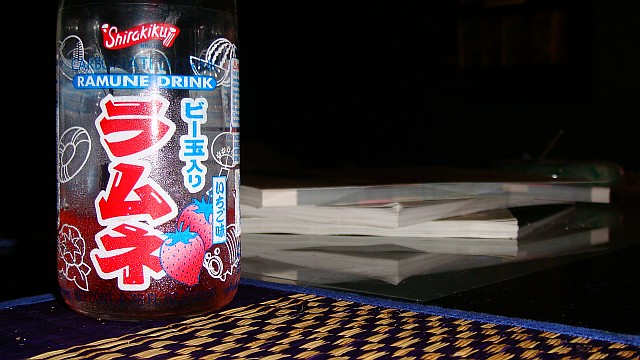This is a detailed and descriptive caption amalgamating the key elements of each provided caption:

In the foreground of the image, a clear bottle of what appears to be an energy drink is prominently featured against a predominantly black background. The bottle, showcasing East Asian characters in red, white, and blue, contains a small amount of red liquid at the bottom and is adorned with a red logo that possibly reads "Shikaku" with "Ramun drink" clearly printed above the symbols. The bottle is decorated with images of strawberries. Beneath the bottle is a brown and black woven checkerboard mat, with a piece of blue tape visible. On the right side of the drink, there is a disorganized stack of books, their pages visible, as they lie in an irregular, overlapping fashion. The combined elements create a visually intriguing scene on what seems to be a dark surface, blending textures and cultural references.